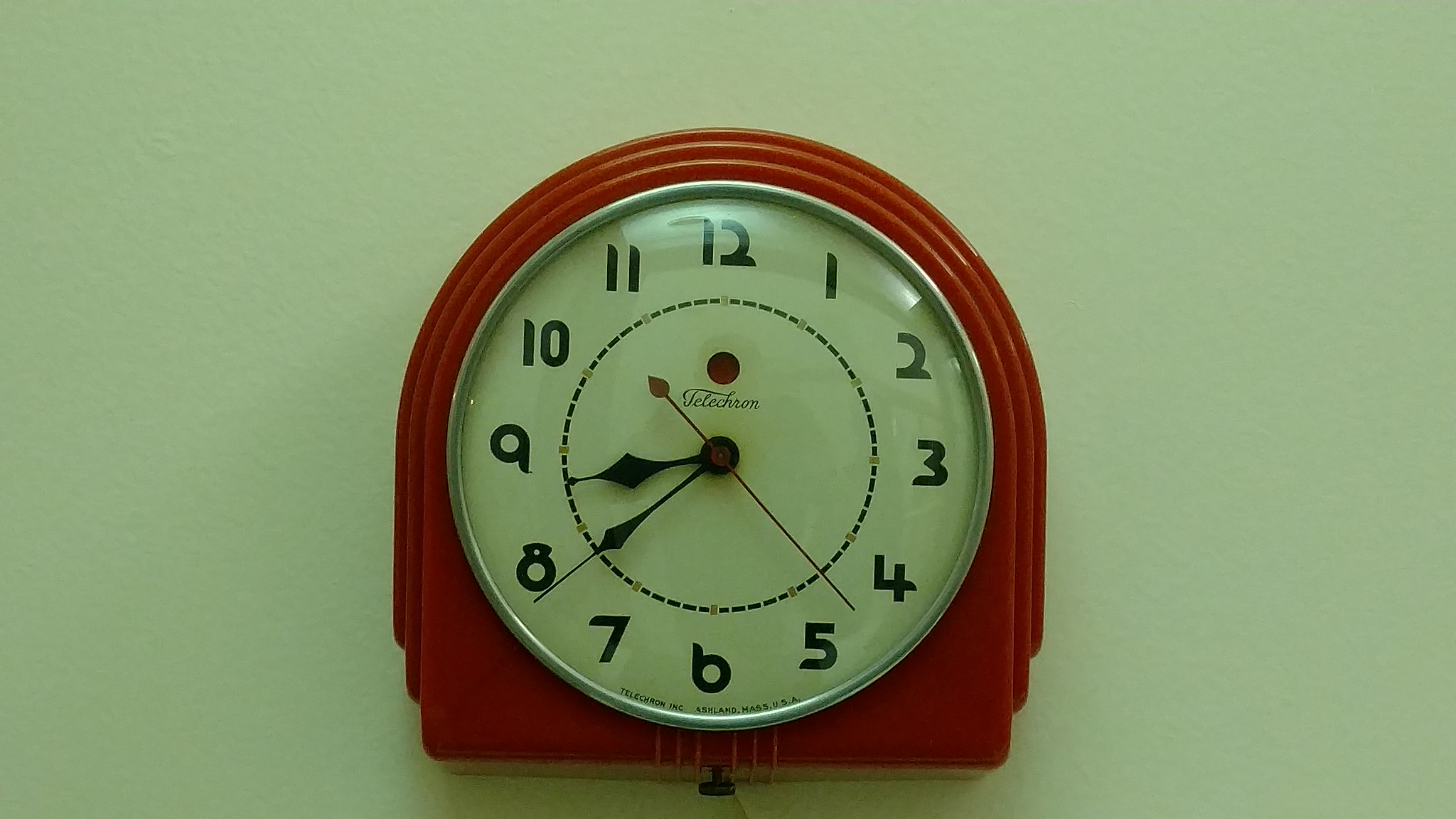This well-lit indoor photograph showcases a high-quality, wall-mounted clock. The clock, crafted from red metal, features a unique flat-bottom semi-circular design. Subtle details, such as the barely legible brand name "TELECHRON" centrally positioned on the clock face, add a touch of sophistication. An intriguing small red dot sits just above the brand name, enhancing its visual appeal.